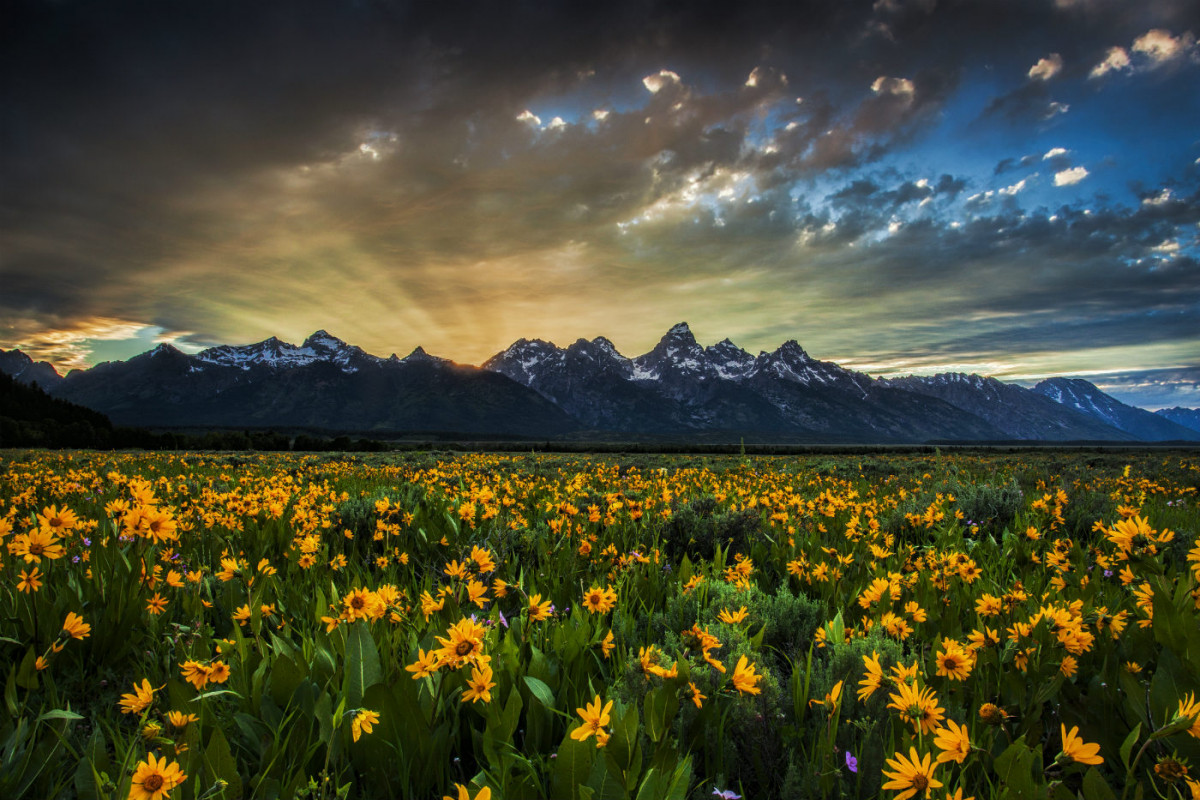This captivating photograph captures a vast field of bright yellow flowers, possibly small sunflowers or yellow daisies, with distinct brown centers. Interspersed among the tall green grass and dominating yellow blooms are delicate, tiny purple flowers, adding a charming contrast. This sea of flowers extends endlessly toward the horizon. In the background, an awe-inspiring range of mountains reaches high into the darkening sky, their towering peaks capped with pristine snow that streaks down their ridges. The sky above is an array of bluish-gray clouds, partially obscuring a blue sky. A sliver of sunlight peeks over the mountaintops, casting golden rays that imbue the scene with hues of yellow, light green, pink, and light blue. The interplay of light and shadow from the setting sun enhances the natural beauty and serene atmosphere of this breathtaking landscape.